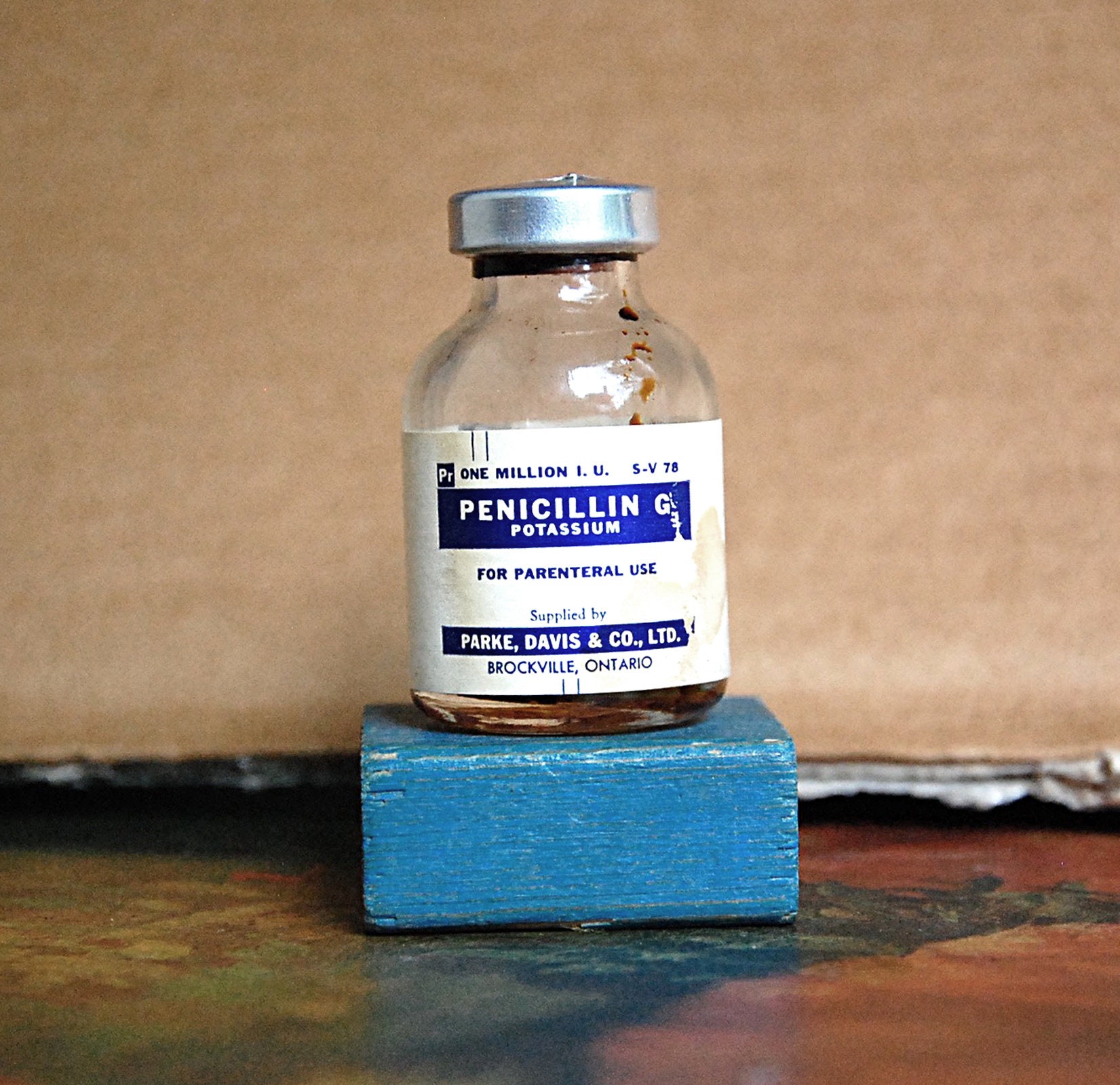This image is a color photograph depicting a vintage glass bottle of penicillin G potassium. The small, clear glass bottle, which has a silver metal cap, rests on a block of light blue painted wood, which fits the base of the bottle snugly. The label on the bottle, now yellowed with age, is primarily white with blue text and a blue rectangle. It reads "PR 1,000,000 IU SV78 Penicillin G potassium for parenteral use, supplied by Park Davis & Co Ltd, Brockville, Ontario." The label shows signs of discoloration and wear, while the bottle itself contains some remaining dark brown liquid at the bottom, visible under the label, and some splatters inside the upper part. The scene is set against a backdrop that appears to be a piece of brownish, cardboard-like material. The surface on which the blue wooden block rests is a floor with a mix of black, greenish, cream, and maroonish-brown colors.